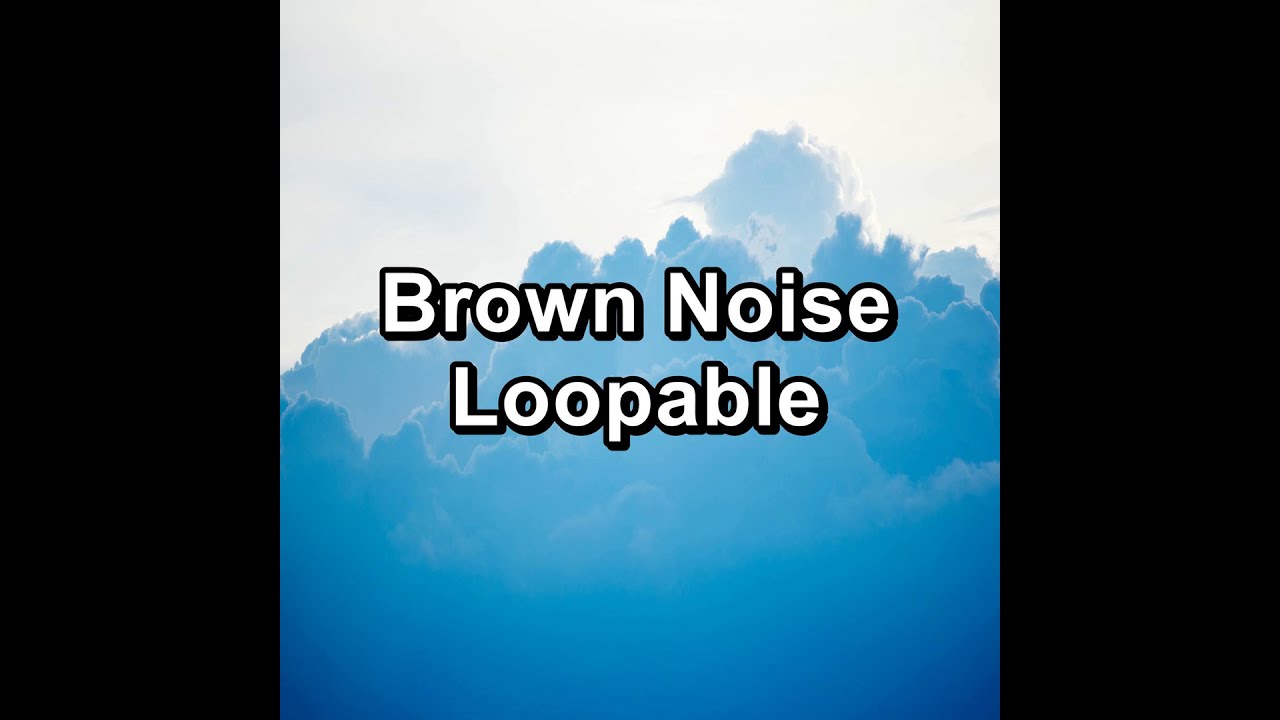The image is a horizontally rectangular thumbnail featuring a photograph of clouds, partially framed by black bars on the left and right sides, which cover about 20-25% of the image's width. In the center, a square section showcases the clouds with a bluish-gray filter, transitioning to a solid gray cloud layer towards the top. The sky above the clouds is white and hazy, creating an ethereal backdrop. Overlaid in the center of the image is white text with a black outline, reading "Brown noise loopable," along with additional mentions of "brown noise." The detailed and descriptive text suggests the image is advertising a loopable brown noise track, emphasizing its soothing, low-frequency sound.